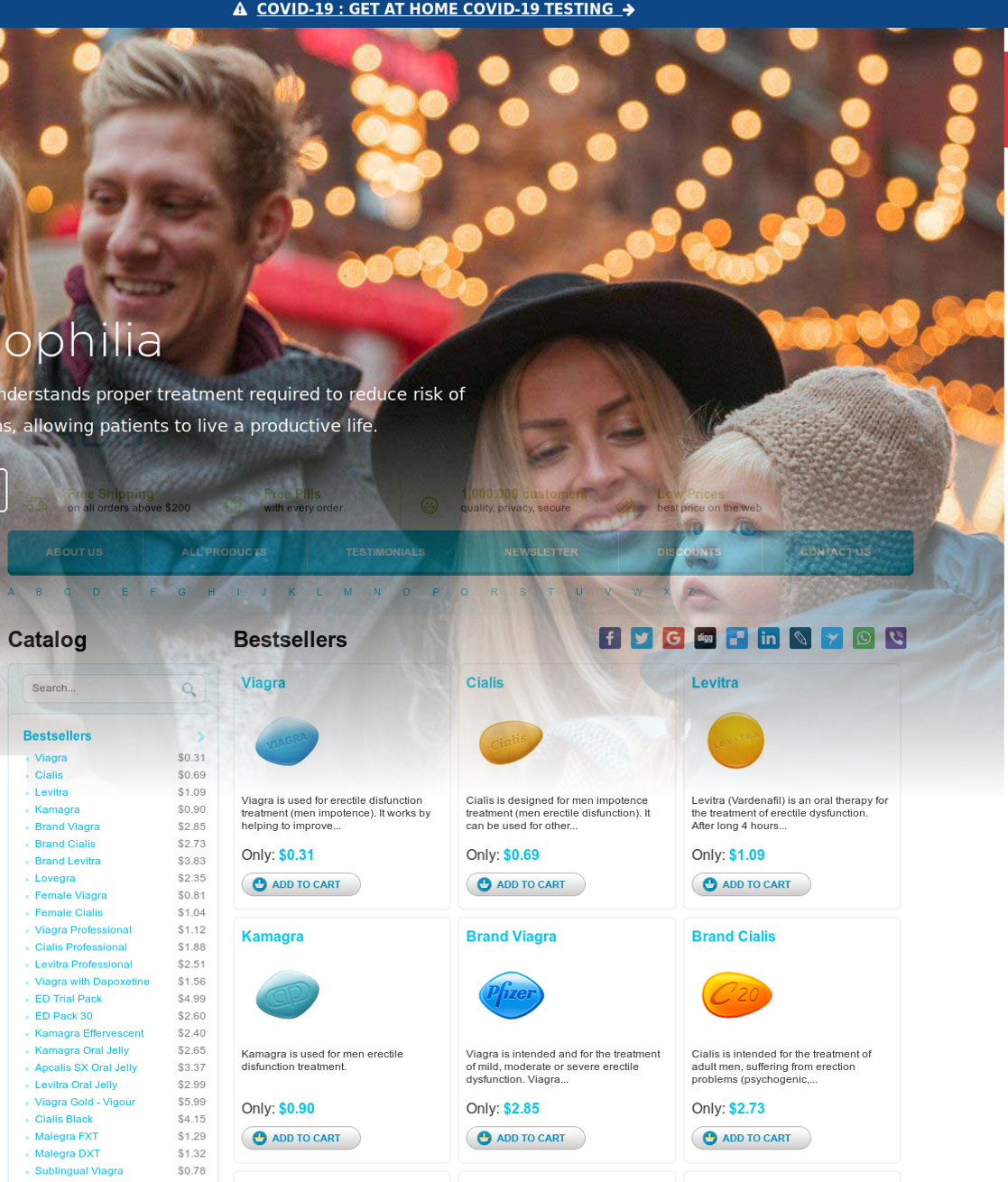The webpage header showcases a prominent blue border with text that reads, "COVID-19: Get At-Home COVID-19 Testing." Below this, there is an image of a family comprising a man, his wife, and their two children, all dressed in heavy winter clothing, including jackets, hats, beanies, and hoodies. The background is intentionally blurred but features numerous yellow Christmas lights and festive decorations, enhancing the holiday atmosphere. Underneath the family photo, there is a blue box followed by several smaller boxes containing brand icons, primarily of social media platforms. The left side of the page includes a sidebar labeled "Catalog," featuring a list of items in blue hyperlinks. Adjacent to this column is another with text in black, although it's too small to read. Additionally, there are images of six different pills on the side, each accompanied by a brief description underneath.